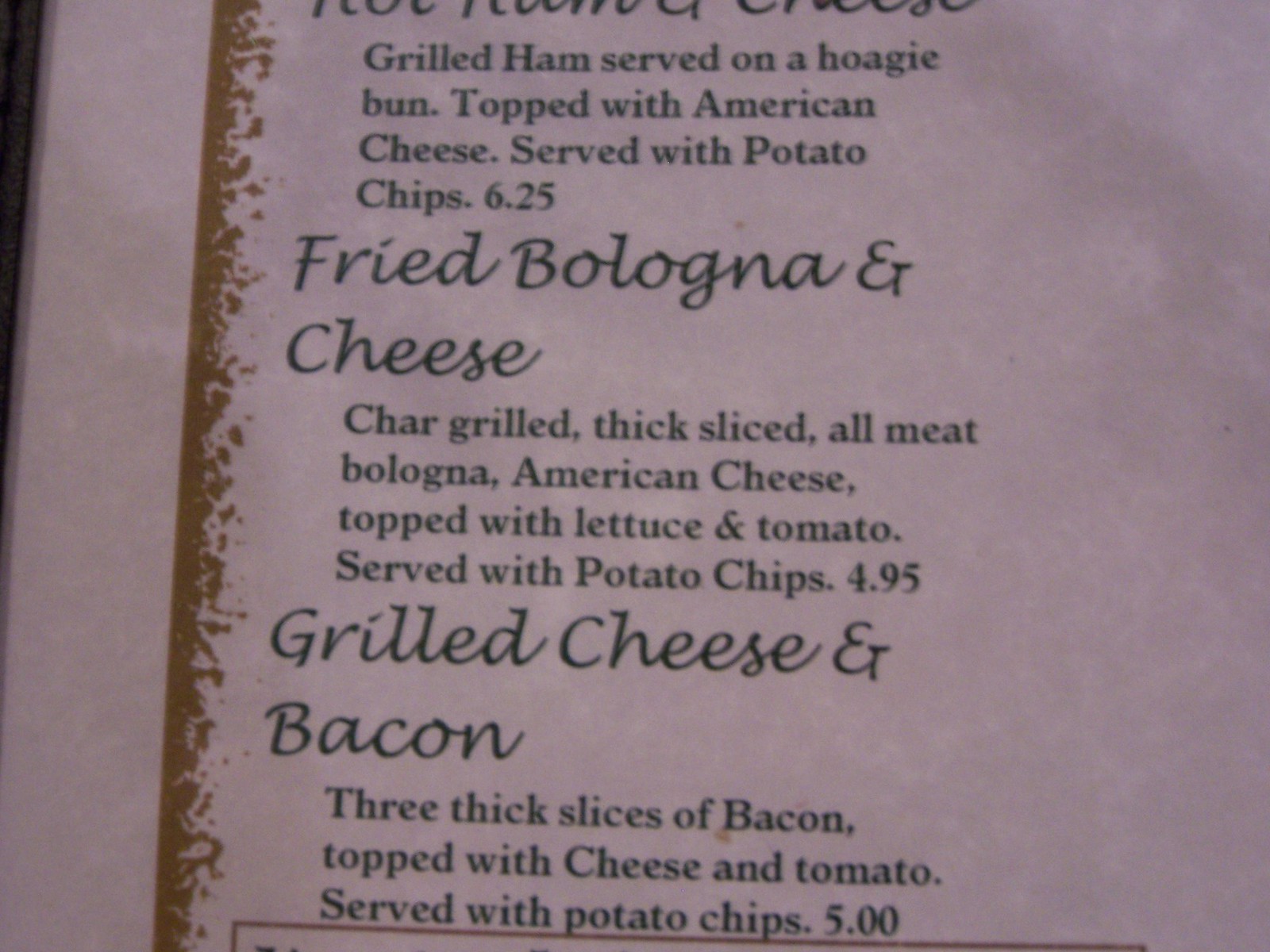In the image, we see a portion of a menu featuring several items, written in a black script font on a white background. Two menu items are prominently displayed. 

The central item, written in a large, elegant script, reads "Fried Bologna and Cheese." Beneath this title, in smaller text, the description details: "Char-grilled, thick-sliced all-meat bologna, American cheese topped with lettuce and tomato, served with potato chips, $4.95."

Below this, another item in a similar large script font is titled "Grilled Cheese and Bacon." Its description reads: "Three thick slices of bacon topped with cheese and tomato, served with potato chips, $5.00."

At the top of the image, though the exact name of the item is obscured, the description remains legible: "Grilled ham served on a hoagie bun, topped with American cheese, served with potato chips, $6.25."